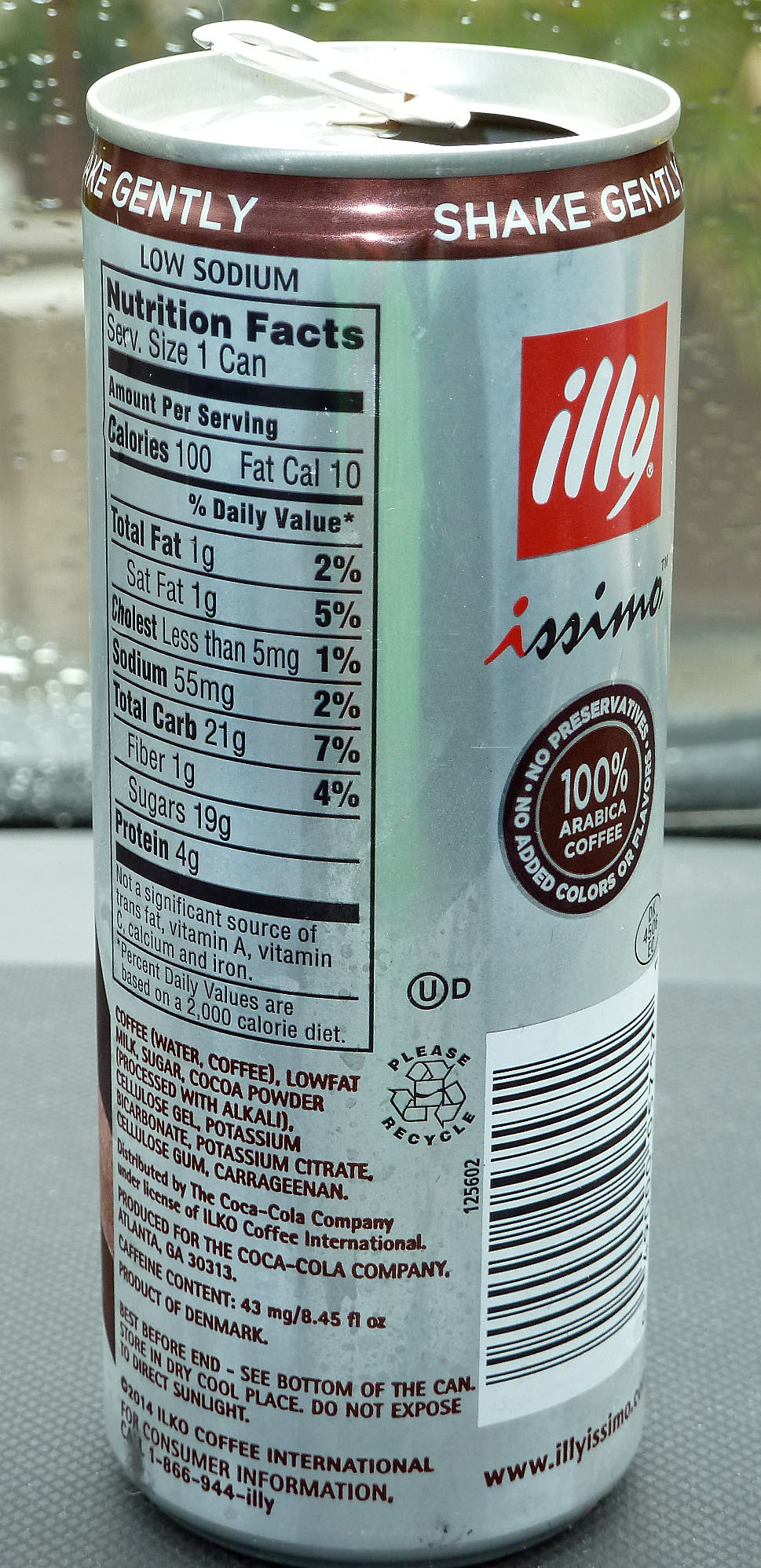The image features a sleek, gray can of ILLY issimo coffee. Encircling the top of the can is a distinct brown strip with the text "Shake Gently." Prominently displayed on the front, the brand name "ILLY" is in bold uppercase letters, with "issimo" elegantly scripted below in cursive. Adjacent to this, a circular label highlights key product attributes: "No Preservatives," "No Added Colors," and "100% Arabica Coffee." Additionally, the can is marked as "Low Sodium" and provides nutritional information on the back, revealing it contains one serving with a total of 100 calories.